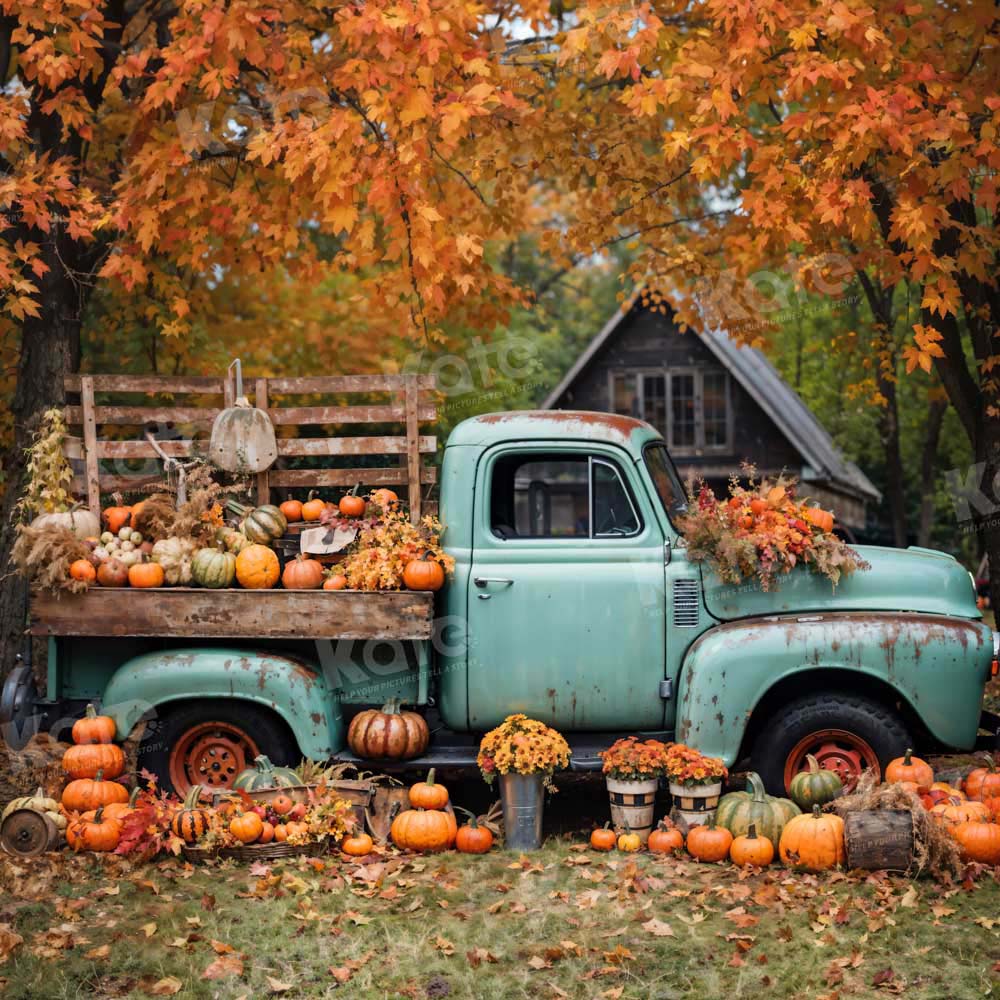Set against the vibrant backdrop of New England in the fall, this captivating image features an iconic late 1940s to early 1950s turquoise, rust-ridden pickup truck brimming with a rich assortment of fall produce. The flatbed is laden with a delightful variety of pumpkins, gourds, and squash in shades of deep orange, green, white, and tan, capturing the essence of an idyllic countryside harvest scene. Surrounding the truck, clusters of potted orange and yellow flowers in both ceramic and metal pots add splashes of color. Fallen leaves carpet the green grass, echoing the hues of the foliage above—trees adorned in stunning autumnal shades of yellow and orange.

Behind the truck, an aging country cottage with a slightly dilapidated roof enhances the rustic charm of the scene. Evergreen trees peek out from behind the cottage, their rich green a striking contrast to the autumnal display. A whimsical touch is provided by a miniature craft gate and decorative pumpkins on the flatbed, while sprays of fall colors and leaves lay scattered across the truck’s hood. This serene, picturesque setting evokes the quintessential charm of a peaceful, run-down village, perfect for a leisurely stroll to buy your fall harvest products.